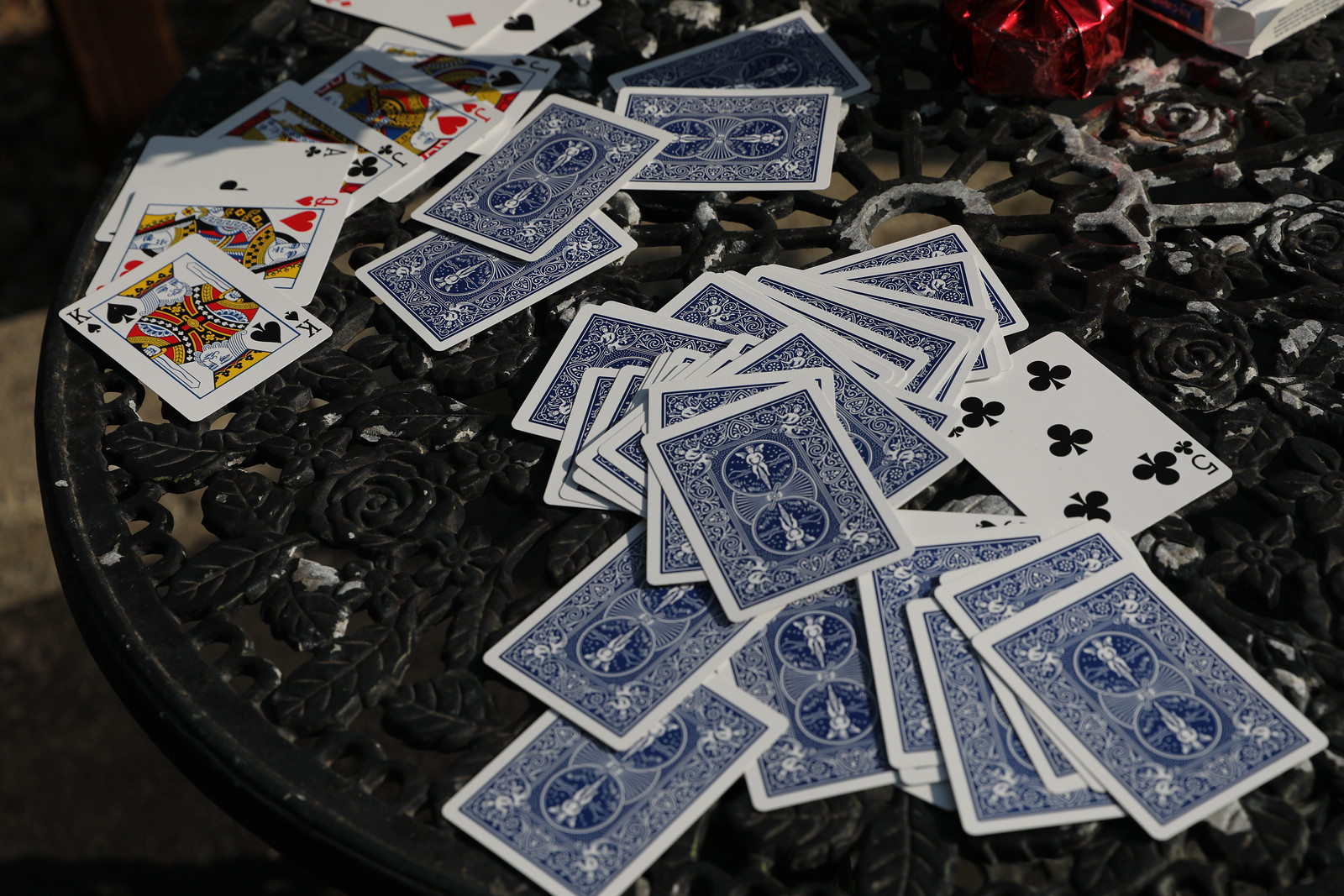The image portrays an outdoor setting during the late afternoon, suggested by the interplay of light and shadows. The photograph features a rectangular patio table with intricate black wrought-iron edges adorned with a swirling rose pattern. The table surface shows signs of slight wear, with areas speckled by a grayish film. In the center of the table is a hole designed to accommodate an umbrella, though it is currently unoccupied. 

Scattered across the table are several Bicycle playing cards. A neat pile of cards lies face down, revealing only their iconic blue back design, with a single five of clubs visible on top. To the upper left section of the table, a variety of cards, including Kings, Queens, Jacks, Aces, and other lesser visible cards, are spread out, some partially cropped out of the shot. A red object, indistinct and placed in the background, adds a splash of color to the scene.